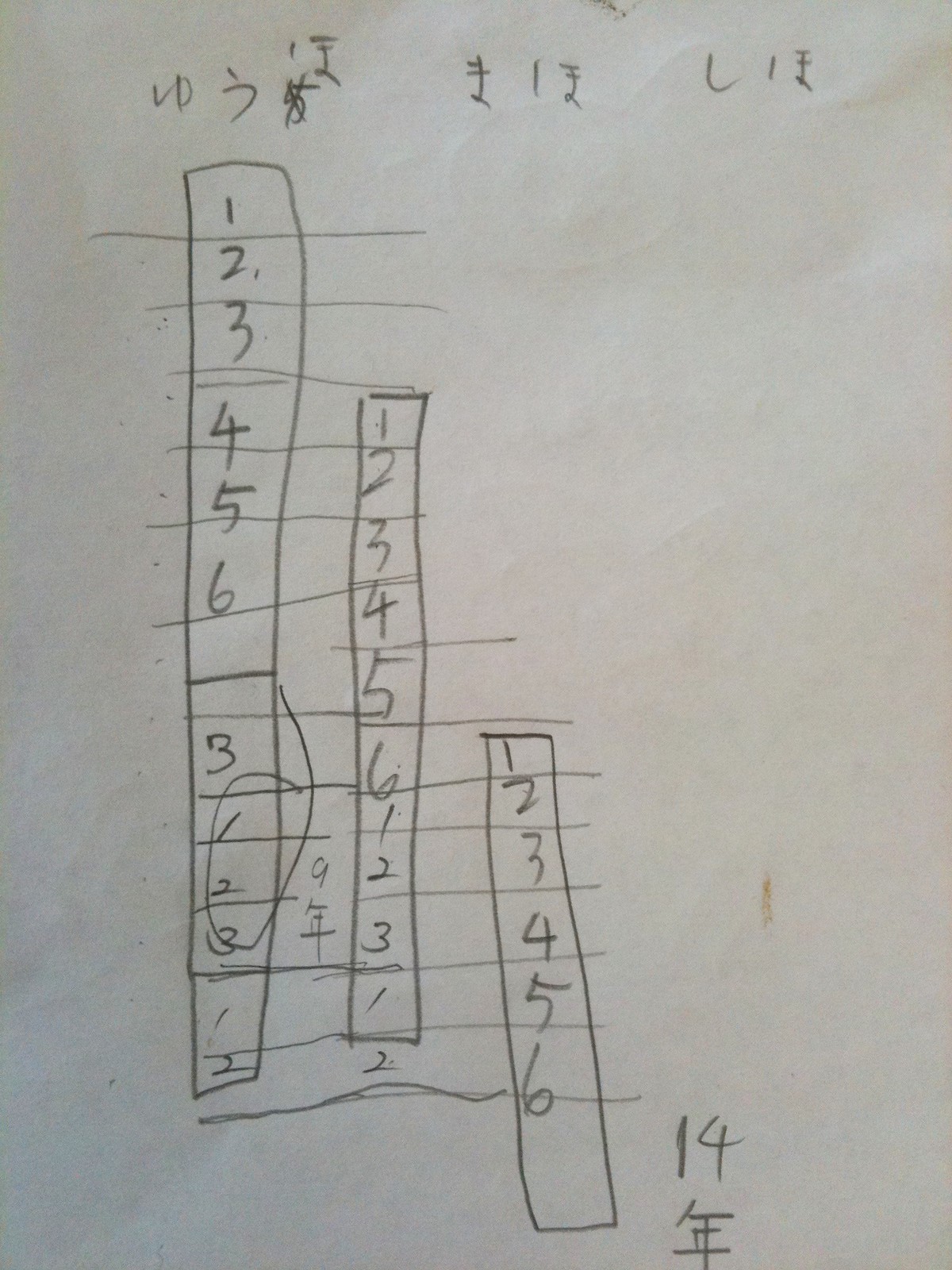In the foreground, the image showcases a piece of paper covered in penciled writings and various Asian characters—likely Chinese, Korean, or Japanese—accompanied by Arabic numerals. The paper features both horizontal and vertical lines creating a grid of rectangular boxes each containing different numbers. 

Specifically, the first vertical column of boxes includes the sequential numbers 1 through 6, and a repeating sequence of 3, 1, 2. Further down, a smaller vertical column repeats the sequence 1 through 6 followed by 1, 2, 3, 1, and 2, with the last number placed just outside of the box. The third vertical column also contains the numbers 1 through 6.

Some horizontal lines span across all three vertical columns, while others cover only one or two columns. In the lower-left corner, the number 14 is prominently displayed above a possible Asian character. The header of the paper is adorned with additional Asian characters possibly as titles or labels.

The overall appearance of the paper is influenced by varied lighting, giving it a white background with subtle hues of blue, light green, purple, and pink, adding depth and dimension to the scene.